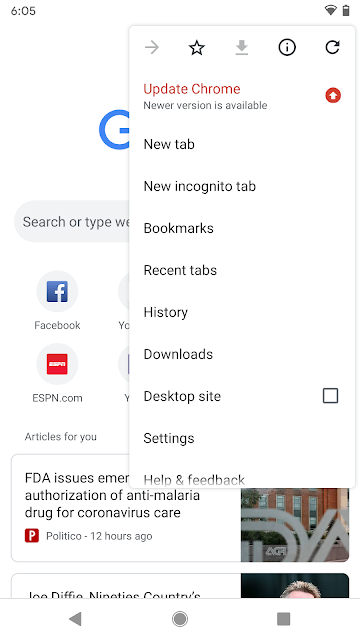Caption: 

A screenshot of a Google Chrome browser on a desktop, featuring a notification indicating the availability of a newer version. The browser interface displays a series of standard menu options, including 'New Tab,' 'New Incognito Tab,' 'Bookmarks,' 'Recent Tabs,' 'History,' 'Downloads,' 'Desktop Site,' 'Settings,' 'Help and Feedback,' and a search bar with the prompt "Search or type URL." Above this menu, there is a series of icons including Wi-Fi, battery, and a download arrow, suggesting system status updates. Notably, the screenshot highlights a recent news article from Politico, reporting on the FDA's emergency authorization of an anti-malaria drug for coronavirus care, which was published 12 hours ago. The interface also shows common website shortcuts such as Facebook and ESPN, alongside personalized article suggestions.